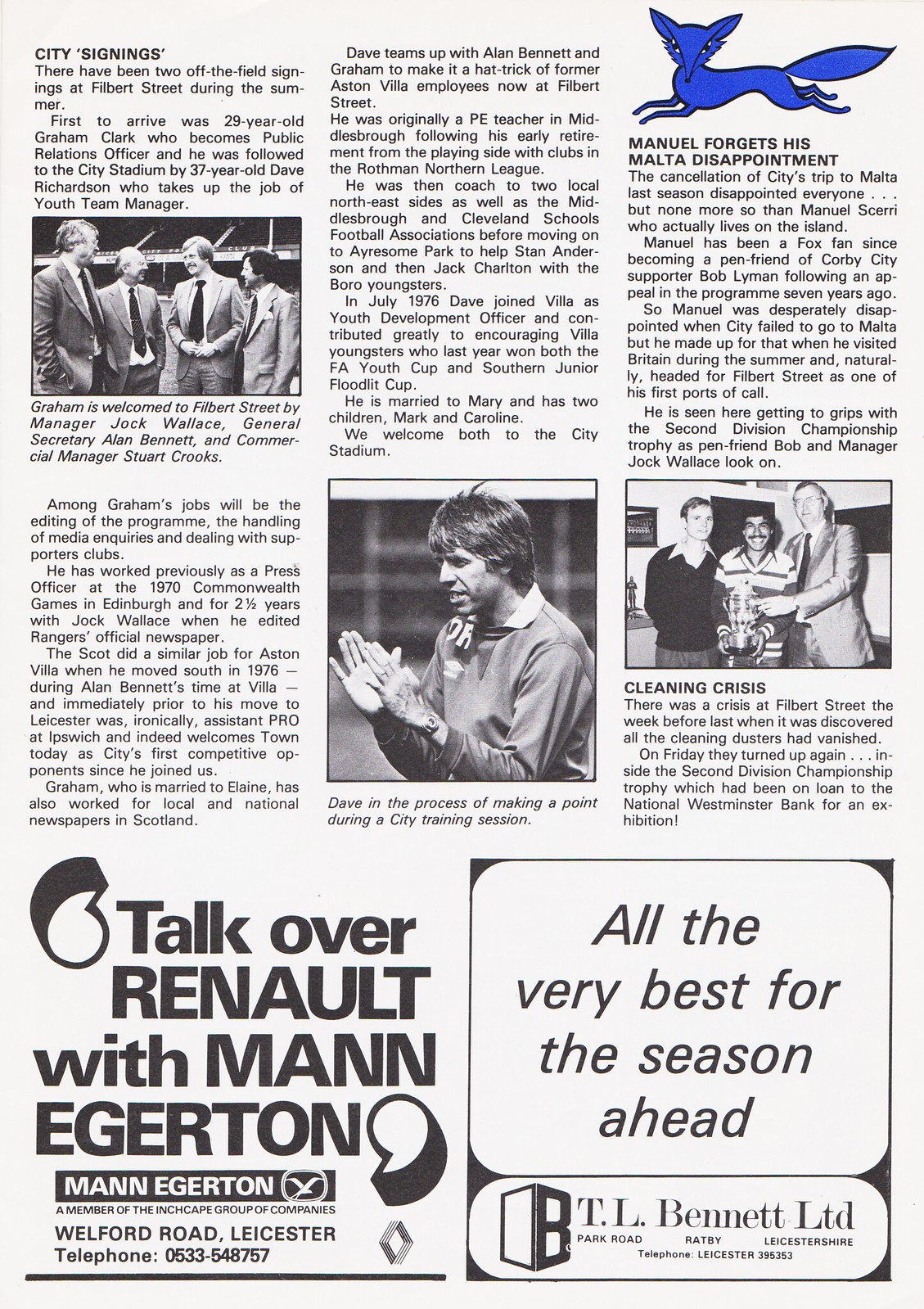This detailed page from an old English football magazine or catalog features a light gray background and is taller than it is wide. It includes three vertical columns of stories discussing signings at Filbert Street, with the main header reading "City Signings." Each column contains black-and-white photographs related to football.

In the first column, there's an image of four men in suits. The caption reads, "Graham is welcomed to Filbert Street by manager Jack Wallace, general secretary Ellen Bennett, and commercial manager Stuart Cripps." The middle column showcases a man in a soccer uniform with his arms raised, captioned as "Dave in the process of making a point during a city training session." The third column starts with a cartoon blue fox and mentions, "Manuel forgets his Malta disappointment." Further down, this column features a photograph of three men hoisting a trophy, though it lacks a caption.

The bottom part of the page is split into two advertisements. On the left, for Mann Egerton in Leicester, it reads, "Talk over Renault with Mann Egerton, a member of the Inchcape group of companies, Welford Road, Leicester, telephone 0533-548-757." On the right, the ad from TL Bennett Ltd. wishes the team success for the season ahead, stating, "All the very best for the season ahead by TL Bennett Ltd, Park Road, Ratby, Leicestershire, telephone Leicester 395-353."